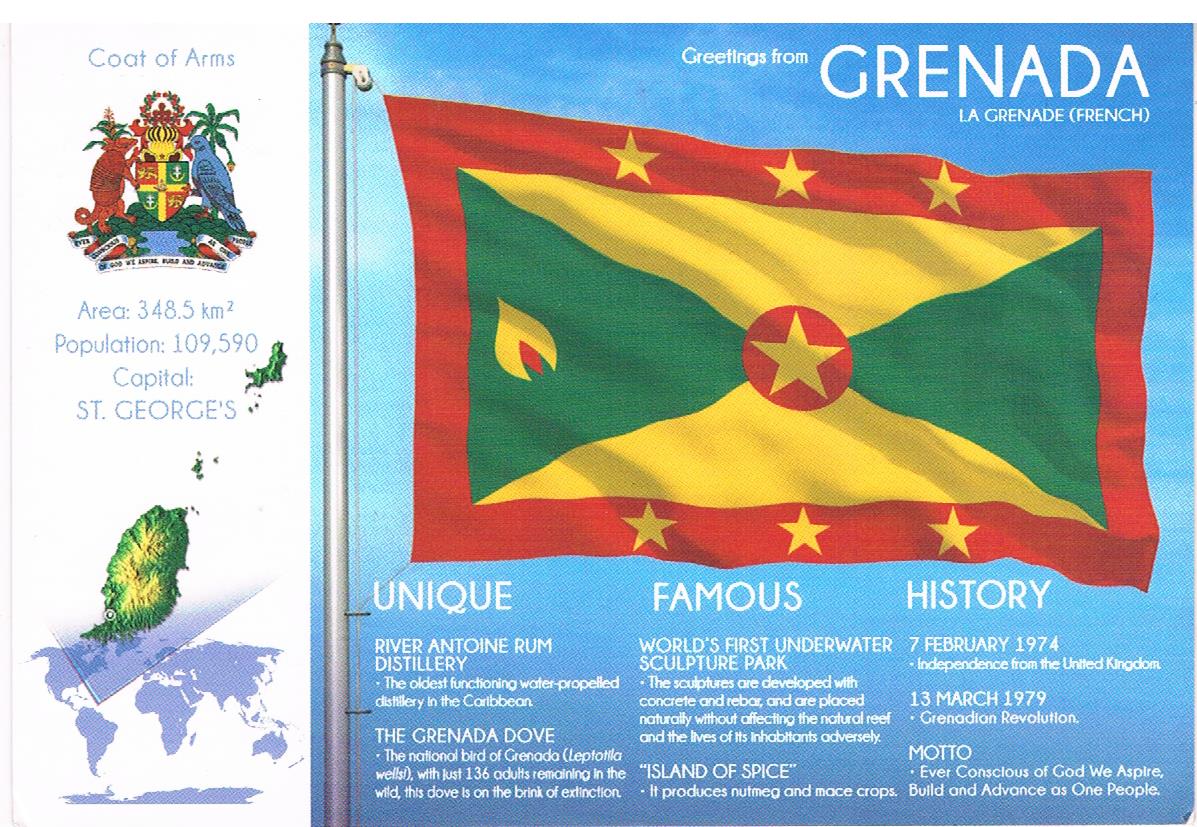This image is designed to resemble a postcard, emphasizing information about the island nation of Grenada in the South Caribbean. On the left edge, a white banner vertically spans the image from top to bottom. At the top, it reads "Coat of Arms," followed by a colorful depiction of Grenada's coat of arms. Below this, in blue text, it lists the area as "348.5 km²" and the population as "109,590." Further down, there's a small green map of the island and text indicating the capital as "St. George's." 

The right three-quarters of the image features a cerulean blue background with Grenada's flag prominently displayed on a pole. The flag comprises a red, yellow, and green color palette, with a central yellow star encircled by red, flanked by yellow and green triangles, and bordered by three yellow stars on both the top and bottom red margins. Above the flag, white text reads "Greetings from Grenada / La Grenade French." Below the flag is a section titled "Unique Famous History" with white text detailing notable points: the world's first underwater sculpture park, Grenada's independence on 7th February 1974 from the United Kingdom, and the Grenadian Revolution on 13th March 1979. It also includes the national motto, "Ever conscious of God. We aspire, build and advance as one people."